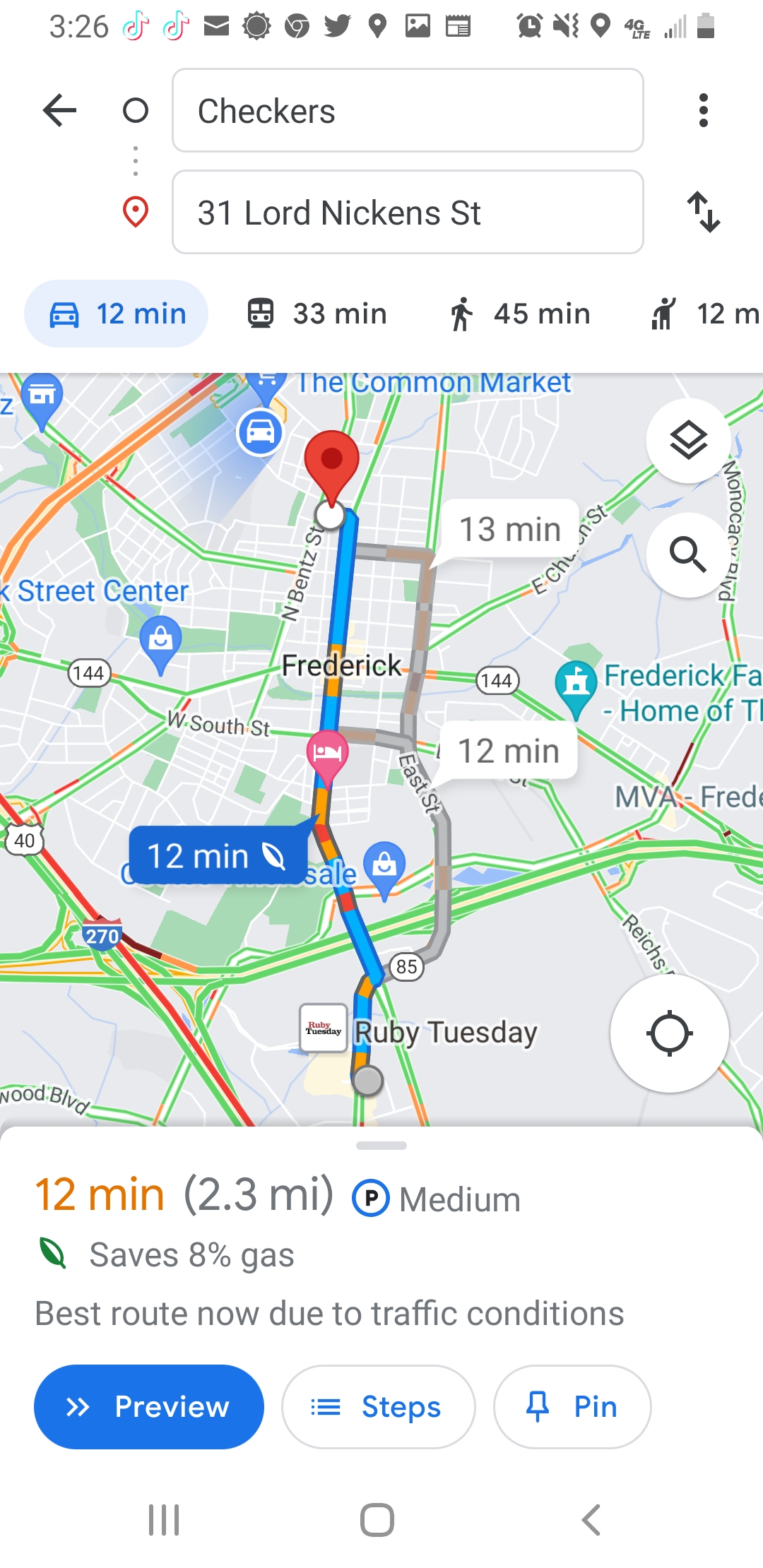The image is a detailed screenshot taken from a smartphone displaying a GPS map of Frederick, specifically highlighting the best route from Checkers to 31 Lord Nickens Street. The map, part of a navigation app, indicates multiple routes with alternate paths shown in gray. The primary route, highlighted for its efficiency due to traffic conditions, spans 2.3 miles and takes approximately 12 minutes by car. Additional transit options show it would take 33 minutes by bus and 45 minutes on foot. Key elements depicted at the top of the phone screen include the time (3:26), various app icons (TikTok, Twitter, Mail, Google Chrome), battery status, and internet connectivity. The map itself features significant landmarks and street names, such as route 270 and the connection to route 40, as well as West-South Street and the Common Market. The image suggests that the highlighted route is optimal for the current traffic situation.